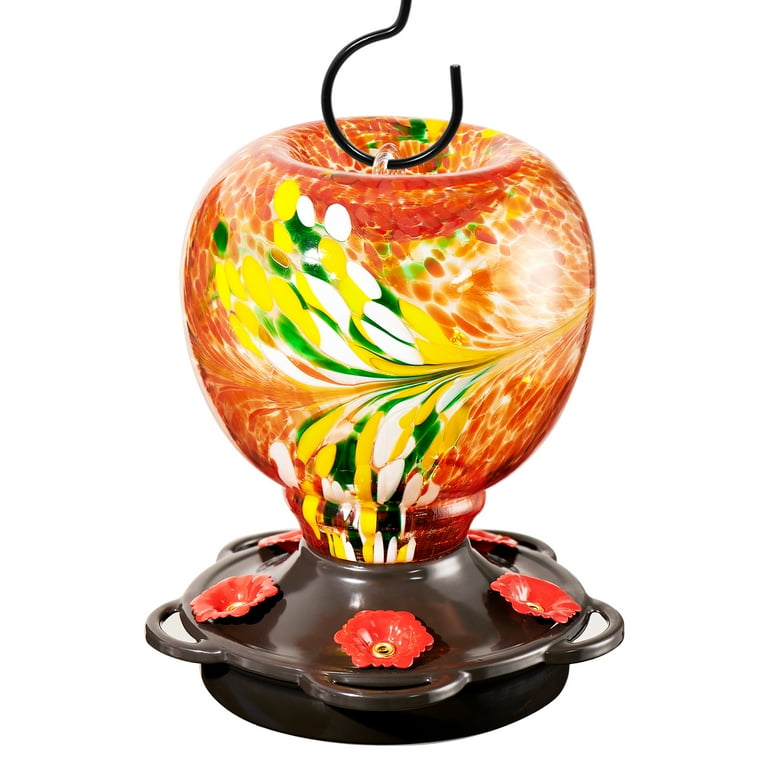The image depicts a strikingly decorative hummingbird feeder, designed to resemble an apple. The feeder hangs from an open-ended black metal hook, which inserts where the stem would be on an apple. The main body of the feeder is a beautifully blown glass dome, showcasing a blend of vibrant colors — red, yellow, green, and white — with a translucent finish and intricate flower designs all around it. At its base, the feeder features a gray circular platform adorned with multiple red and yellow-centered flowers. These flowers serve as perches and access points for hummingbirds to drink the nectar. The base's metallic, flower-like structures and additional upside-down U-shaped gray perches provide stable landing spots for the birds. The entire setup is against a plain white background, enhancing the vivid colors and artistic details of the feeder.